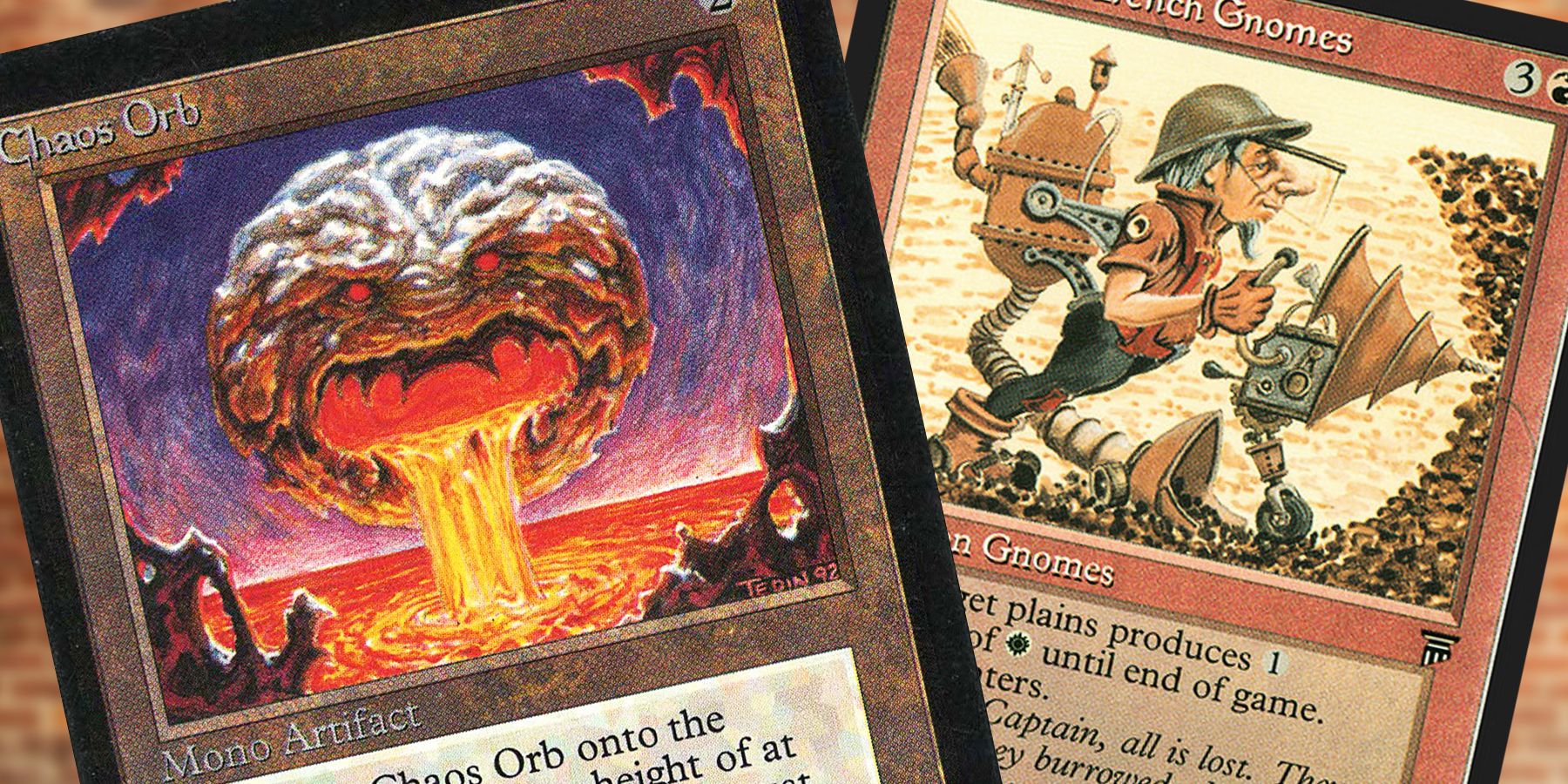This detailed photo showcases a close-up of two tabletop game playing cards: the one on the left — titled "Chaos Orb" — and the one on the right centered around "Gnomes." Both cards dominate the frame, leaving slight hints of a brown table in the background corners. The Chaos Orb card is depicted with a dark, menacing planet featuring an angry face, lava pouring from its mouth, and fiery red eyes, all set against a purplish-pink backdrop. It is labeled as a mono-artifact, although the detailed text beneath is partially obscured. The card has a brown background and a black border. The Gnomes card on the right, which has a salmon-pink background and a white number "3" in the top right corner, features an industrial scene: a gnome, equipped with a steampunk-style mechanical drill, operates the device against a hard surface, emitting an aura of mechanical ingenuity. This card too has a black outer edge, and the artwork suggests that gnomes play a role in production until the end of the game.